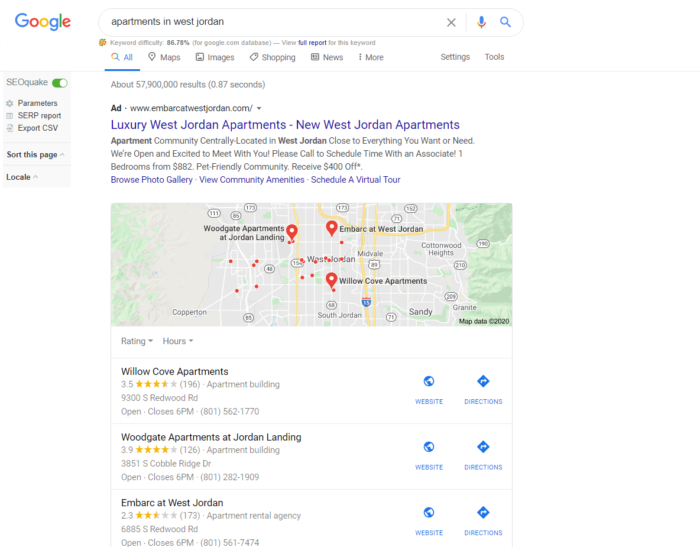Detailed Caption: 

The screenshot shows Google search results in the upper left corner with the familiar Google colors—blue, red, yellow, and green. The search bar contains the query "apartments in West Jordan," and the page is currently on the "All" tab. Other tabs available include "Maps," "Images," "Shopping," "News," and "More." 

The search has generated approximately 57.9 million results in 0.87 seconds. The first listing is a paid advertisement for luxury apartments in West Jordan with the headline "Luxury West Jordan Apartments | New West Jordan Apartments." The ad links to the URL "embarkatwestjordan.com" and promotes centrally located apartment communities that are close to essential amenities. It invites potential tenants to call or schedule a visit, highlighting various features like one-bedroom apartments starting at $882, a pet-friendly environment, a $400 discount offer, a photo gallery, community amenities, and virtual tour options.

Below the ad, there is a horizontally elongated map displaying three apartment complexes: Woodgate Apartments at Jordan, Embark at West Jordan, and Willow Cove Apartments. Willow Cove Apartments has a rating of 3.5 stars based on 196 reviews and is located at 9300 South Redwood Road. The office hours indicate that it is open and closes at 6 p.m. The phone number listed has a Utah area code (801).